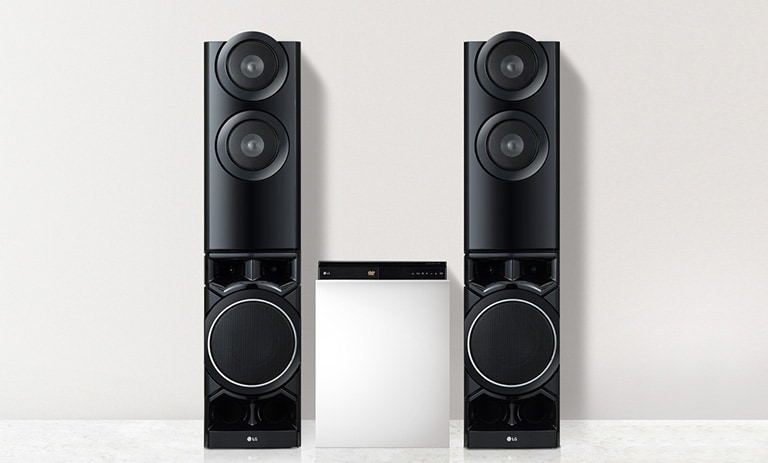In this computer-generated photograph, two tall, rectangular black sound speakers are set symmetrically against a plain white wall and white floor, lending a contemporary and minimalistic feel. Each speaker features two round speaker heads stacked at the top, below which sits a larger round speaker with a distinctive white circular trim. Just above and below the larger speaker, pentagon-shaped speakers add visual intricacy. Positioned centrally between the two speakers is a modern, metallic-looking device with a white body and a black top, which hints at some kind of control or enhancement unit for the audio system. The black top of this middle device features a gold emblem, adding a touch of elegance to the clean and sleek setup.